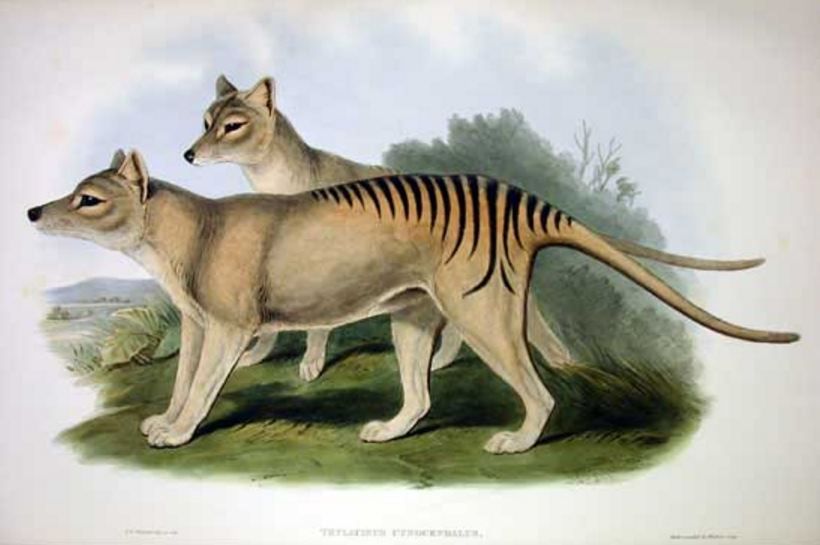The image depicts a detailed painting with a predominantly white background and grey borders. Central to the composition are two Tasmanian tigers standing on a green grassy terrain, facing left. Both animals are seen in side profile, with one slightly behind the other, revealing mostly its shoulders and head. The tigers are light brown with grey tones and distinguishable black stripes running from mid-back to the tail. Above them, a light blue sky stretches across the top of the painting, with large trees forming a backdrop. The lower edge of the painting features faint, small black text that is too small to read. The scene captures the tigers in their natural habitat, showcasing fine details like the grassy surface and the bush-inflected landscape that extends into a distant valley. Colors in the painting include shades of white, light blue, gray, green, brown, tan, and black, contributing to a serene yet intricate portrayal of the animals and their environment.